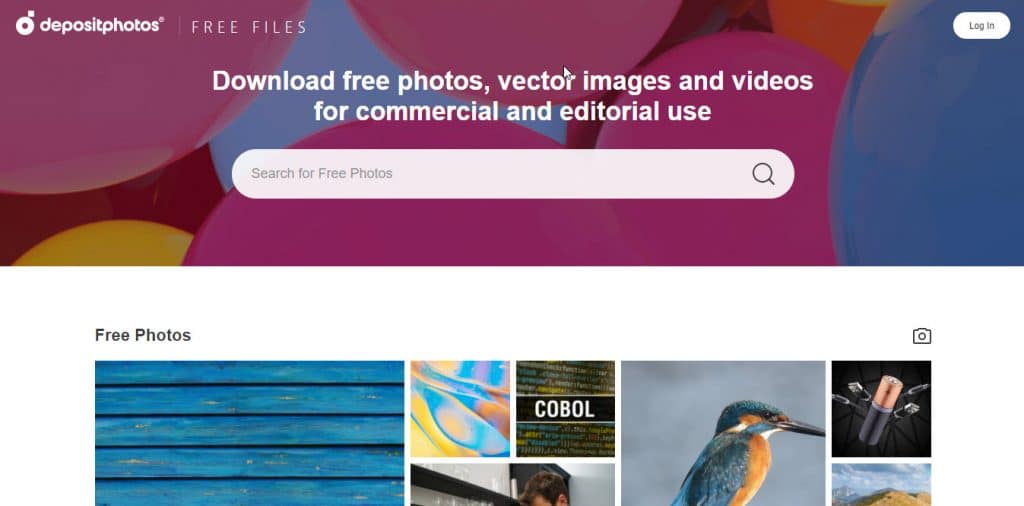This image depicts a webpage interface with a visually engaging layout. At the top of the page, a large rectangular banner showcases a vibrant mix of colors with parts of balls in hues of purple, blue, and yellow. In the top left corner of this banner sits a small white circle with a purple dot inside. Adjacent to this circle, the text "Depositphotos" is prominently displayed, followed by "Free Files" to the right.

On the top right corner of the banner, a "Login" button stands out with black letters on a white background. Central to the banner is the text highlighting the primary offer of the site: "Download free photos, vector images, and videos for commercial and editorial use." Directly beneath this message, a white search bar with the text "Search for free photos" offers users the ability to search the site. Both the left and right ends of the search bar feature a magnifying glass icon, indicating the search functionality.

Below this main banner, there is a white space that leads to another rectangular section containing a selection of various photos. At the top left of this section, the words "Free Photos" are written in black. Directly below this text is an image of a blue-colored side of a house or a similar structure. To the right of this image are four more pictures arranged in a row: the first appears to feature an animal, the second includes the text "cobble," the third showcases a bird with a distinctive blue head, blue wings, a brown chest, and a black beak, and the fourth depicts what seems to be a battery with a copper top and a black bottom. Beneath the battery image, there is a landscape photograph, adding to the collection of diverse visuals on the page.